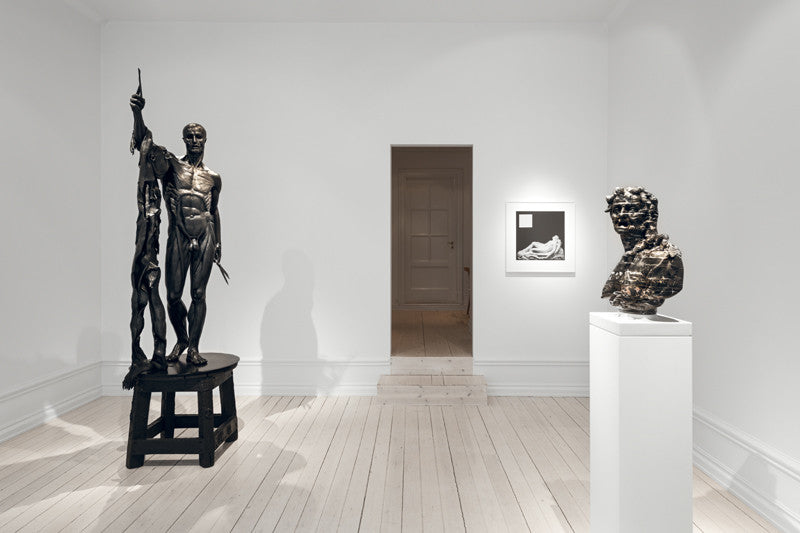The image depicts a brightly lit white room, likely part of a museum or gallery, with a light wood-colored floor that gives the space an airy feel. On the left side of the room stands a larger-than-life, dark metal statue of a man seemingly without skin, posed as if holding up a branch or stick. The statue is perched atop a small black table or stool. To the right, there is a bronze-looking bust of a person, gazing towards the camera, mounted on a white pedestal. The wall behind this artwork is adorned with a framed picture, depicting a somewhat ambiguous figure lying down, against a dark background. Nearby, a narrow doorway opens up to reveal another room with a brown door further in the background, adding to the sense that this space might have once been part of an older home. The overall ambiance is minimalistic, emphasizing the displayed art pieces.